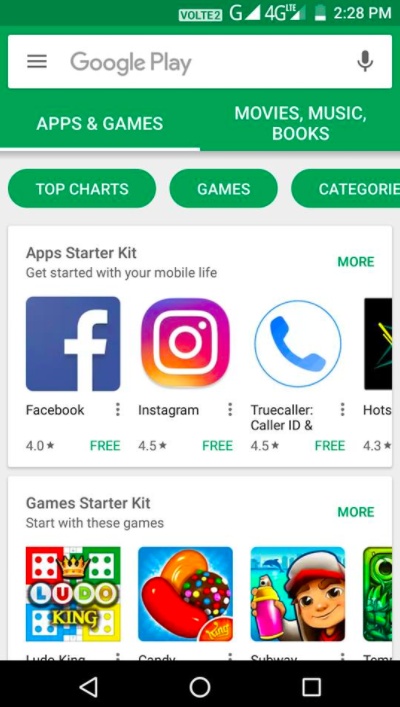This image is a photograph of a cell phone screen displaying the Google Play Store interface. At the top, a green header features a white rectangular search bar labeled "Google Play" with a microphone icon beside it. Just below, a navigation menu lists options: "Apps & games" on the left, and "Movies, Music, Books" on the right. Further down are several elongated menu buttons, including "Top Charts," "Games," and "Categories."

The first section highlighted is an "App Starter Kit" titled "Get started with your mobile life," featuring app icons for Facebook, Instagram, Truecaller, and a partially cut-off fourth app. Below each icon, the app names are displayed in text alongside their star ratings: Facebook (4.0), Instagram (4.5), and Truecaller (4.5).

Following this, a "Game Starter Kit" section invites users to "Start with these games," showcasing small thumbnails of different games. Three game icons are visible, but the fourth is cut off, obscuring both the icon and its name. Overall, the image provides a comprehensive view of the Google Play Store layout and its categorized app offerings.